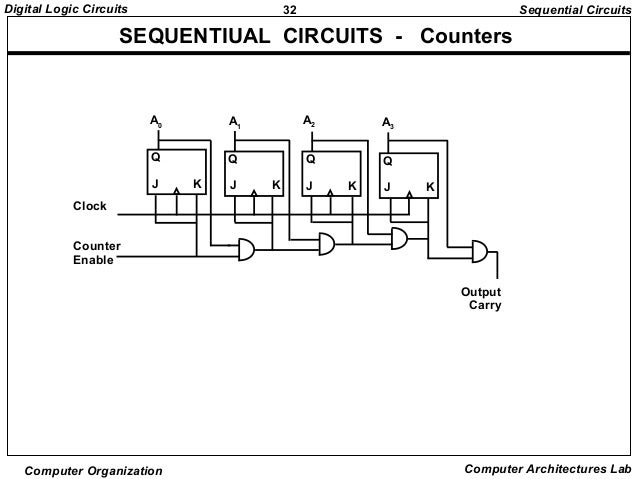This black and white image is a detailed diagram titled "Sequential Circuits - Counters." It's presented on a white background. The top left corner features the text "Digital Logic Circuits" followed by the number 32, possibly indicating a page number. To the right, it reads "Sequential Circuits." Below the title, a thick black line separates the header from the main illustration, which consists of a series of interconnected squares.

In the center of the diagram, a group of four labeled squares is displayed. These squares, marked as A0, A1, A2, and A3 from left to right, are part of the sequential circuit being depicted. Each square contains the letter Q in the upper left corner, a J in the lower left corner, and a K in the lower right corner, suggesting the J-K flip-flop components of the circuit.

The left side of the diagram begins with the word "Clock," and beneath it are the words "Counter Enable" and "Output Carry," indicating the flow and control mechanisms within the circuit. Arrows connect these labels to the boxes, highlighting the sequential progression through the circuit.

The bottom left corner of the diagram reads "Computer Organization," while the bottom right corner is labeled "Computer Architectures Lab," signifying the educational or research context of the illustration.